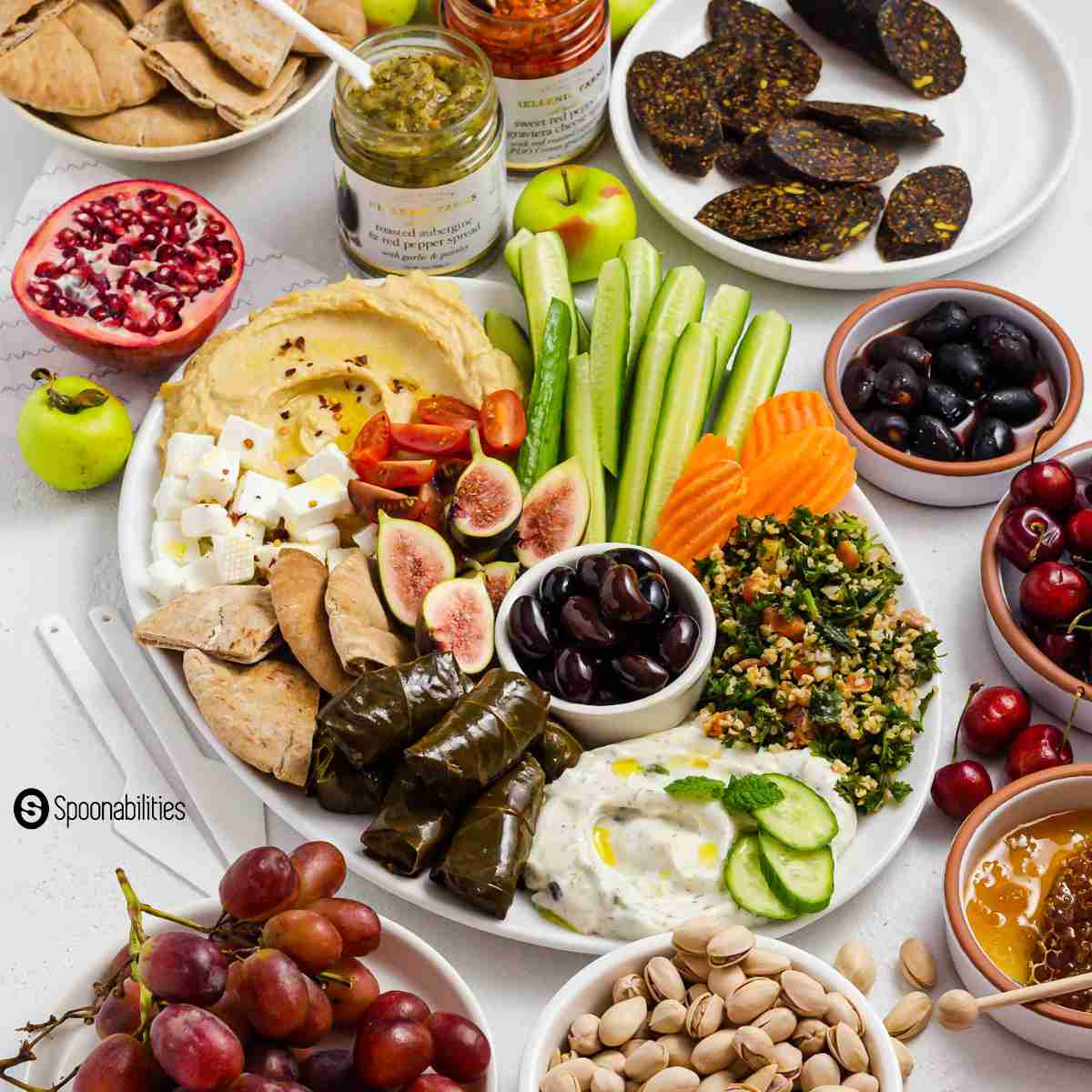This detailed color photograph showcases an inviting spread of Mediterranean-inspired dishes meticulously arranged on a solid white marble table adorned with dark gray squiggle lines. At the center of the composition lies an oval white platter bursting with an array of fresh raw vegetables, including spears of cucumbers, carrots, halved cherry tomatoes, and figs, surrounded by cubes of white feta cheese. The platter also features a small bowl of black olives, hummus, and a dollop of tzatziki sauce topped with cucumber slices. 

To the top left, a round white porcelain bowl is filled with triangular cut pita bread. Adjacent to it are two clear jars, one with a green pesto sauce and the other containing a red sauce, flanking a green apple marked with brown spots. Nearby, a white shallow dish holds dark red blood sausage with yellow spots. 

Around the central platter, other delicacies are scattered, including a half pomegranate, clusters of red grapes, a bowl of fresh cherries with a few spilled out, and a dish of pistachios. There are also dolmas, some reddish brown sausages, a bowl of honey with a wooden dipper, and additional olives interspersed throughout. 

On the bottom left of the image, the word "Spoonabilities" accompanied by an S logo can be seen in black text, blending into the realistic and representational style of the photograph.